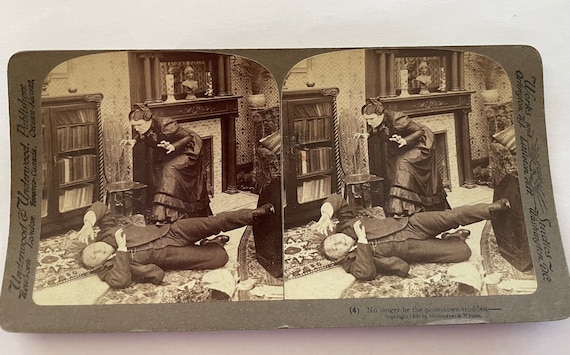This image is an old stereographic reel from the 1800s, designed for use with stereographic glasses to create a 3D effect. The reel features two identical black and white images placed side by side in a wide horizontal rectangular format, with the top edges slightly curved. The scene depicted appears to be taken from an old play and takes place in an elegantly furnished living room with a bookshelf, fireplace, and candles in the background.

In the images, a woman, dressed in a floor-length gown with her hair styled in a bun, is crouched down with both hands extended like claws, seemingly about to attack a man. The man, dressed in a tuxedo suit, has fallen to the floor and is shielding his face with his arms as if to protect himself from her. The pictures are set against a dark gray to almost brown board with nearly illegible black text around the edges. Below the images, there is a small number "4" enclosed in parentheses, whose significance remains unclear.